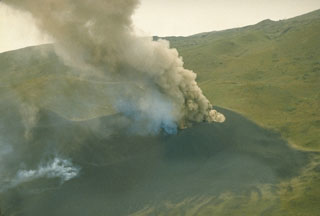The photograph depicts an erupting volcano in a low-resolution image, likely a still frame from an old video or screenshot. Taken from an aerial perspective, possibly from a helicopter, it showcases a vast, green mountainous landscape with no visible inhabitants. In the center, large, thick plumes of dark gray smoke billow aggressively into the sky, fanning out towards the top left of the photo. To the left, there are indistinct shapes that could be coastal waves, adding to the scene's rugged, untamed nature. The sky in the background is a dull gray, devoid of clouds and any hint of blue, enhancing the dramatic and somewhat desolate atmosphere of the volcanic eruption. There is no text cluttering the image.